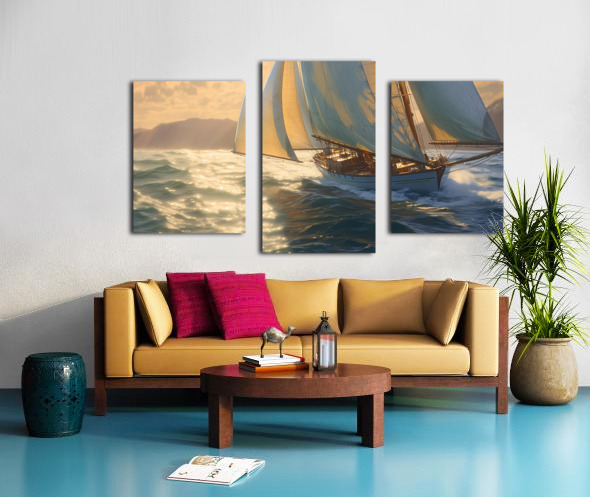The image depicts a well-lit lounge room with beige light grey walls and a polished shiny floor in a light blue, sky blue hue. Central to the room is a modern, mid-century style three-seater sofa with a wooden frame, featuring yellow foam-filled cushions and armrests. The sofa is adorned with four matching gold-yellow pillows and two contrasting bright pink ones. 

In front of the sofa, there is a small circular wooden coffee table, on which three stacked books support an upright camel figurine, alongside an old-fashioned hurricane lamp. On the floor in front of the coffee table rests an open book. 

To the left of the sofa and coffee table is a ceramic pot, while to the right and slightly behind the sofa is another pot containing a plant with long, spiky green leaves. Behind the sofa, three vertically arranged paintings form a triptych depicting a sailboat on choppy waters under a golden beige sky.